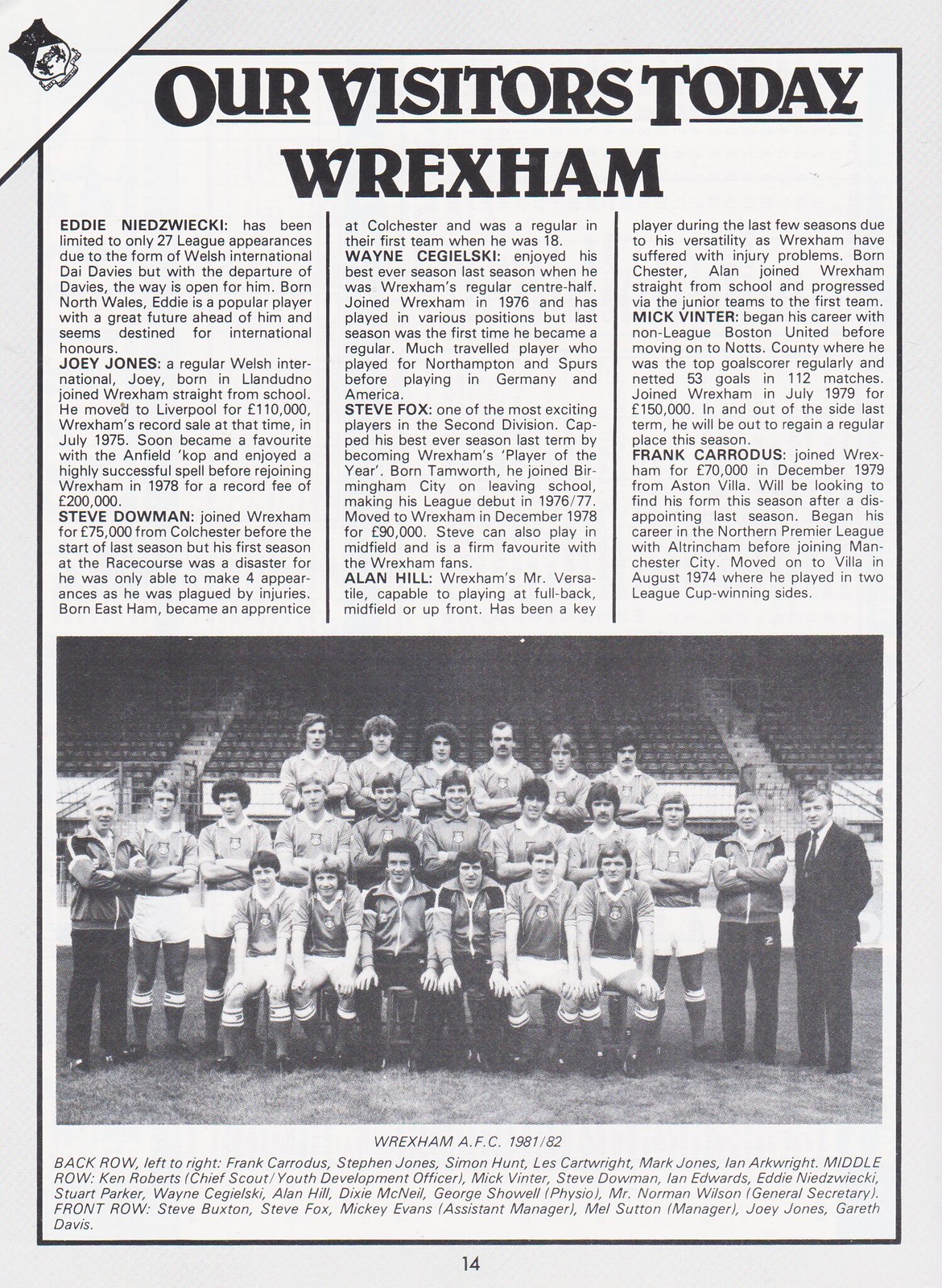This is a black-and-white scan of page 14 from a vintage soccer program featuring the Wrexham AFC team from the 1981-82 season. At the top, bold, underlined text reads "Our Visitors Today, Wrexham." The upper half of the page is split into three text columns, each with headers such as Eddie Nidwitzki, Joey Jones, and Steve Dallman, detailing player names and brief biographies. For example, it notes Eddie Nielsen’s limited appearances due to the dominance of Welsh International Dye Davies, and Joey Jones’ welcome status as a Welsh International. The bottom half features a grayscale photograph of the Wrexham team, showcasing players, coaches, and their distinctive vintage hairstyles, including shaggy hair, mustaches, sideburns, and a few curly afros. The photograph is captioned "Wrexham AFC 1981-82," and lists the names of all pictured individuals. The entire article is bordered by a black line, giving it a classic newspaper feel.